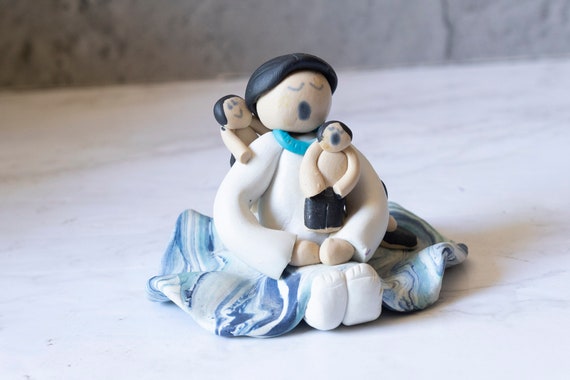The image depicts a rustic, handcrafted clay statue of a woman in traditional attire, seated on a light-colored tiled floor against a backdrop of gray stone or tiled walls. The woman, with black hair and closed eyes, appears to be either yawning or singing, her mouth open. She wears a white dress with a flowing blue skirt and a blue collar-like necklace. Two children with short black hair accompany her; one child, also with closed eyes and open mouth, sits on her lap without a shirt but dressed in black shorts. The other child, smiling with open eyes, leans over the mother's shoulder, similarly shirtless but wearing black shorts. The statue's simplicity gives it a hobbyist or arts-and-crafts feel, rather than a high-art piece. This charming, intimate scene evokes a sense of closeness and maternal care.